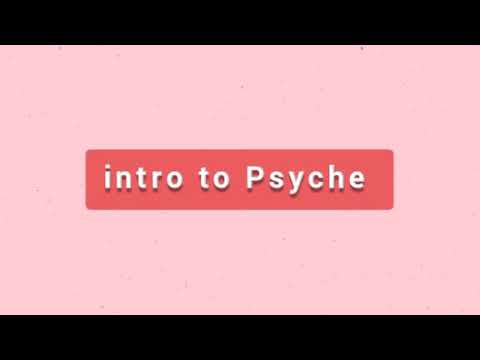The image features a simplistic and easy-to-read design, giving it the appearance of a title or introductory slide, possibly from a presentation or a cover page. It has a light pink background adorned with two thick black horizontal bands at the top and bottom. Dominating the center of the image is a coral-red rectangular box. The box, which spans about four inches in width if the total width is approximated to six inches, contains the text "Intro to Psyche" written in white letters. Notably, the word "Psyche" starts with a capital 'P', while the rest of the text is in lowercase. The font choice is a modern sans-serif, adding a trendy touch to the overall design.